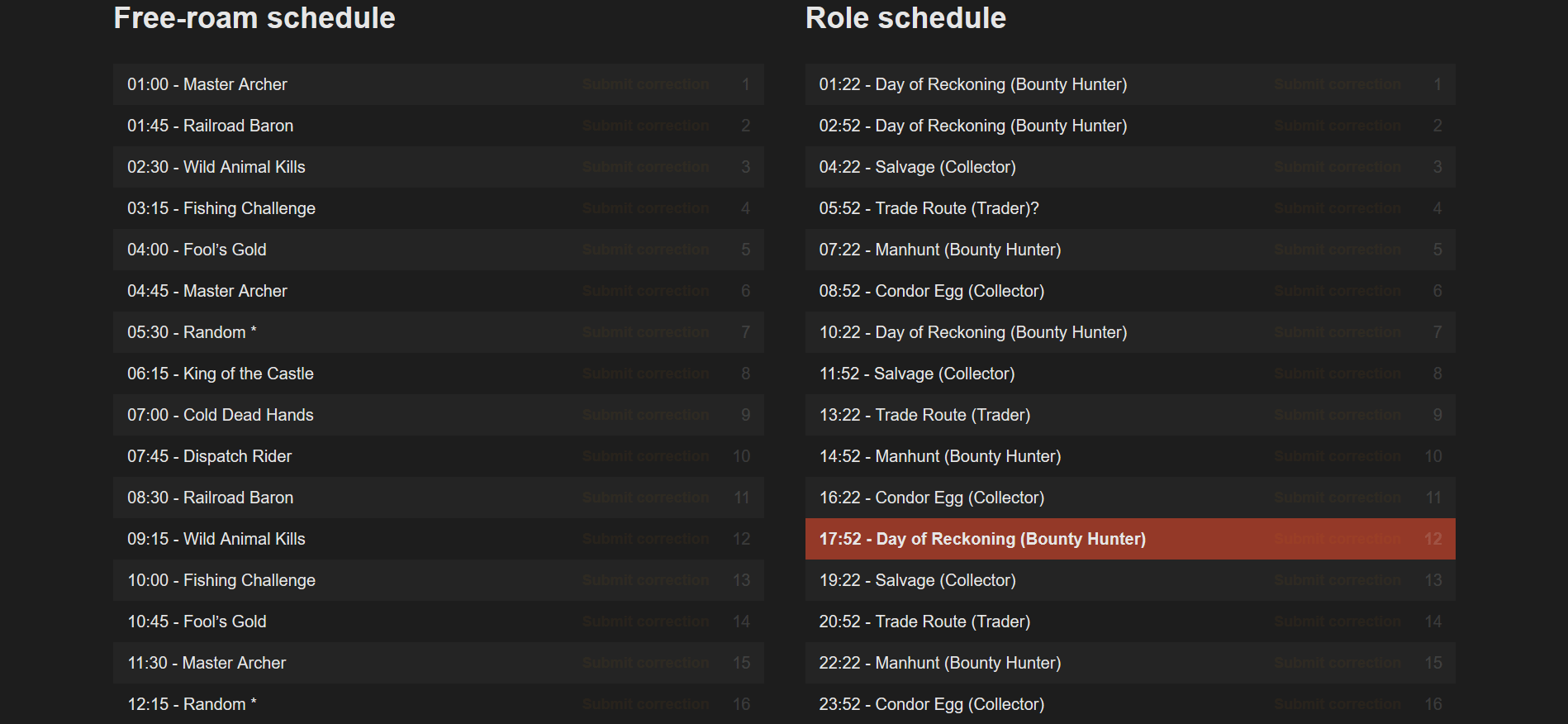This screenshot captures a desktop website interface with a predominantly black background, accented by white text. The highlighted section features an orange banner for emphasis. The layout consists of two vertical columns labeled as rows. The first column is titled "Free Roam Schedule" and lists various activities and their corresponding times. The activities include:

1. Meteor Archer - 1:45 
2. Beans (illegible text)
3. Wild Animal Kills - 2:30
4. Fishing Challenge - 3:15
5. Fool's Gold - 4:00
6. Master Archer - 4:45
7. Random - 5:30
8. King of the Castle - 6:15
9. Cold Dead Hands - 7:00
10. Dispatch Rider - 7:45
11. Railroad Baron - 8:30
12. Wild Animal Kills - 9:15
13. Fishing Challenge - 10:00
14. Fool's Gold - 10:45
15. Master Archer - 11:30
16. Random - 12:15

The second column is titled "Enrolled Schedule" and starts with "Day of Reckoning (Bounty Hunter)" at 1:22.

The text appears somewhat difficult to read due to the quality of the screenshot, but this extensive schedule allows users to plan participation in various activities throughout the day.